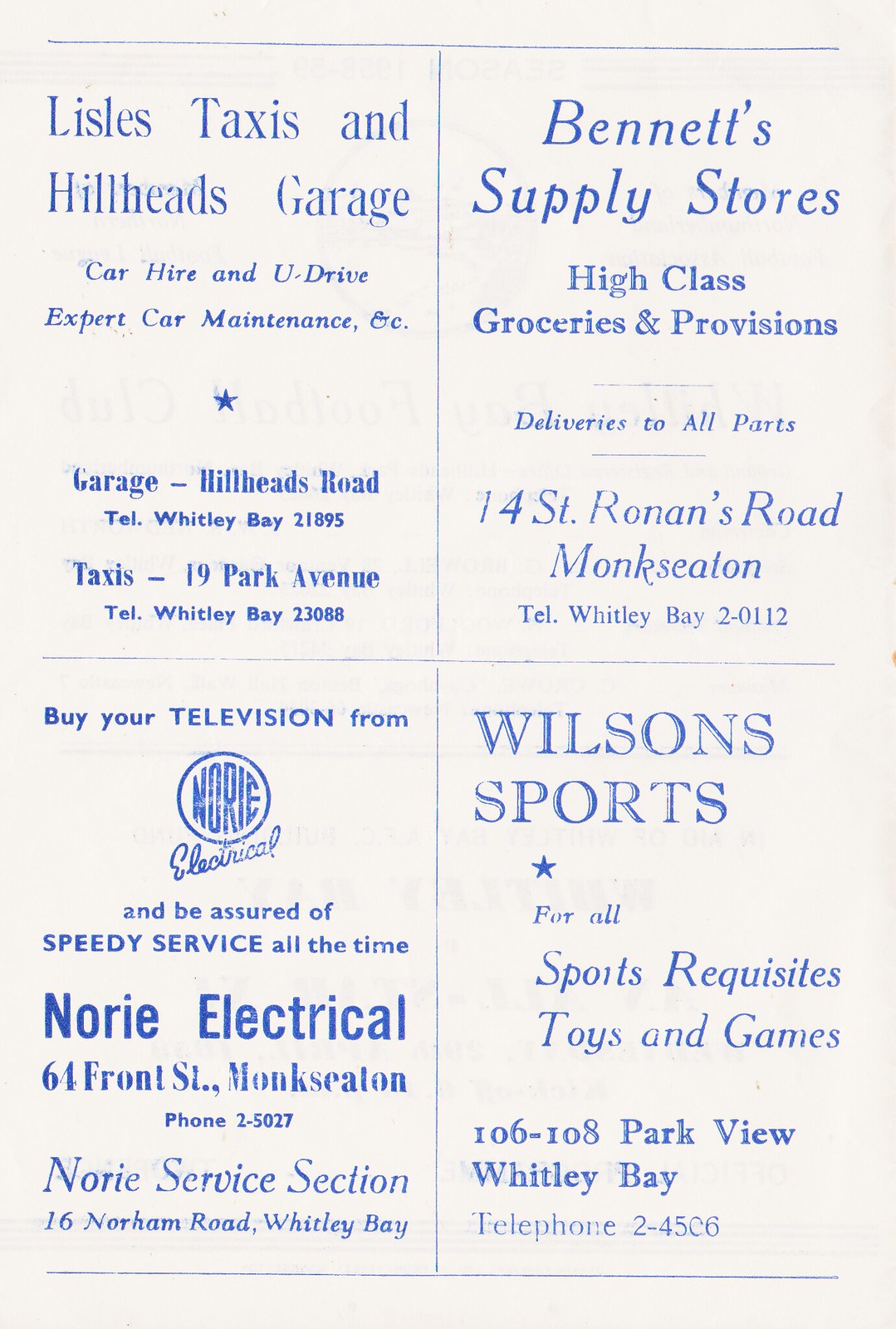**Promotional Flyer with Business Listings**

This visually appealing promotional flyer is displayed with medium blue text, divided into four distinct sections by a bisecting cross, creating a neatly organized 2x2 grid layout. Each section contains an advertisement for a local business, complete with detailed information.

**Upper Left:**
**Lyle's Taxis and Hillhead's Garage**
- **Services:** Car Hire and U-Drive, Expert Car Maintenance
- **Addresses and Contact:**
  - **Garage:** Hillhead's Road, Telephone: Whitley Bay 21895
  - **Taxis:** 19 Park Avenue, Telephone: Whitley Bay 23088

**Upper Right:**
**Bennett's Supply Stores**
- **Tagline:** High Class Groceries and Provisions, Deliveries to All Parts
- **Address:** 14 St. Ronan's Road, Monk Seaton
- **Phone:** Whitley Bay 2-0112

**Lower Left:**
**Norrie Electrical**
- **Tagline:** Buy Your Television from Norrie Electrical and Be Assured of Speedy Service All the Time
- **Addresses:**
  - **Main Store:** 64 Front Street, Monk Seaton, Phone: 25027
  - **Service Section:** 16 Norham Road, Whitley Bay

**Lower Right:**
**Wilson's Sports**
- **Tagline:** For All Sports Requisites, Toys, and Games
- **Address:** 106-108 Parkview, Whitley Bay
- **Phone:** 2-4506